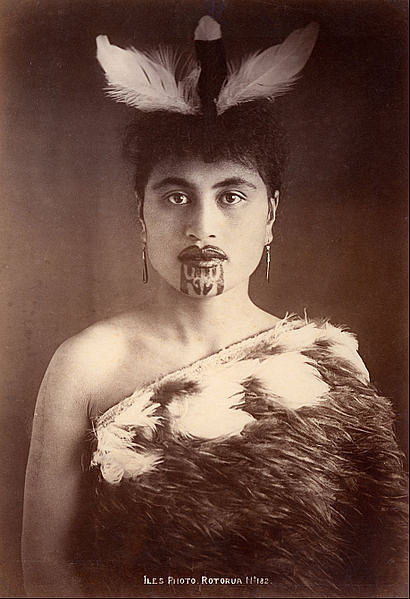In this striking black and white photograph, a tribal woman with an intense gaze looks directly into the camera, framed against a dark background. Her thick, black curly hair is adorned with feathers—three prominent ones on top, with the middle feather being black tipped with white, flanked by white feathers. She wears long, dangling earrings that brush against her neck. The woman's face is marked by distinct tattoos: her lips are artfully decorated and the design elegantly extends to her chin in a swirling pattern with straight edges, giving the illusion of makeup. Her expressive, bushy eyebrows add further character to her visage.

She is draped in a thick fur garment that appears brown with white spots near the top, leaving one shoulder uncovered in a traditional style. Around her neck, a small cap like an adornment rises in a column, complementing her elaborate headdress. Despite the black and white nature of the photo, the texture of her garb hints at a rich, earthy palette. At the bottom of the image, there is small, hard-to-read writing that seems to say "I-L-E-S photo, Rutoro Haza," adding a hint of mystery to her enigmatic presence.